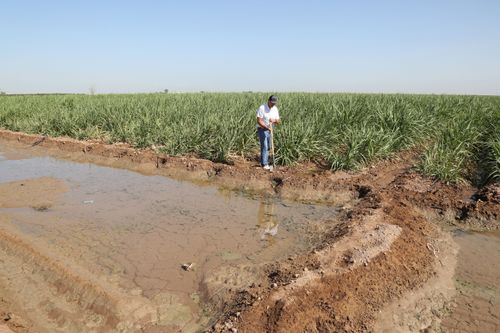This color photograph, likely taken in the Imperial Valley of California, captures a vast sugarcane field stretching to the horizon under a clear, light blue, cloudless sky. In the foreground, there is a notable irrigation ditch, or filtration pond, characterized by its raised dirt berms, filled with accumulated groundwater. Central to the image stands a man, wearing a white short-sleeved shirt, blue jeans, and a black baseball cap. Leaning on a shovel, he appears to be an irrigation expert tending to the ditch, which features small holes along the wall for water drainage from the field. The field itself consists of diagonal rows of green sugarcane plants with long leaves, growing out of reddish-brown dirt that contrasts with the vibrant greenery. The dirt and water-filled areas hint at an intricate irrigation and water filtration system essential for nourishing the crop. In the far distance, faint silhouettes of farm structures or utility poles might be visible against the clear sky, adding depth to the serene agricultural landscape.